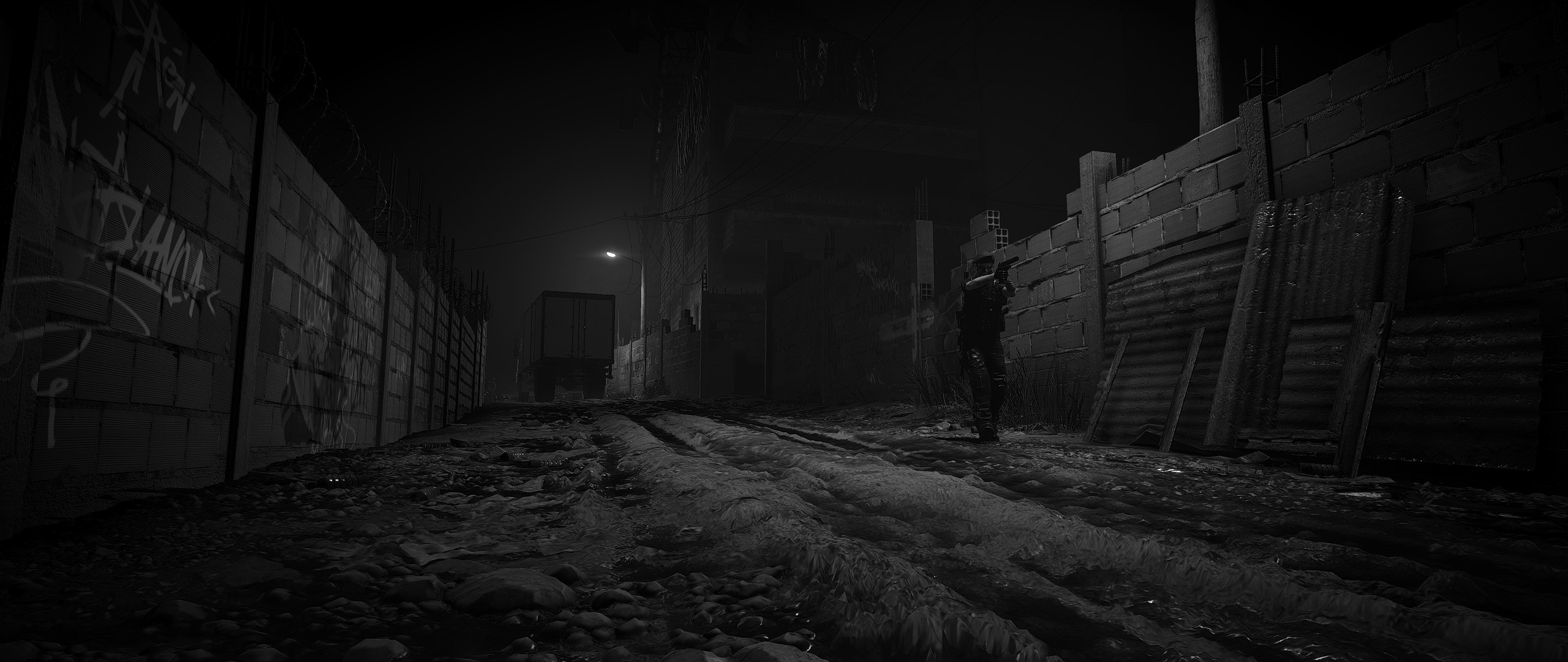In this black and white nighttime photograph, we find ourselves in a bleak alleyway with high brick walls on either side, adorned with graffiti and various objects propped up against them. The ground is a rugged, dirt path strewn with debris, enhancing the gritty atmosphere. Dominating the shot is a lone individual, walking towards the right, seemingly in a uniform that resembles military attire, with a gun pointed straight ahead, adding a tense and ominous feel to the scene. In the far distance, beyond the man, stands a large delivery truck with its back closed and a single streetlight casting a solitary beam of light, piercing through the darkness and partially illuminating both the truck and the distant path.